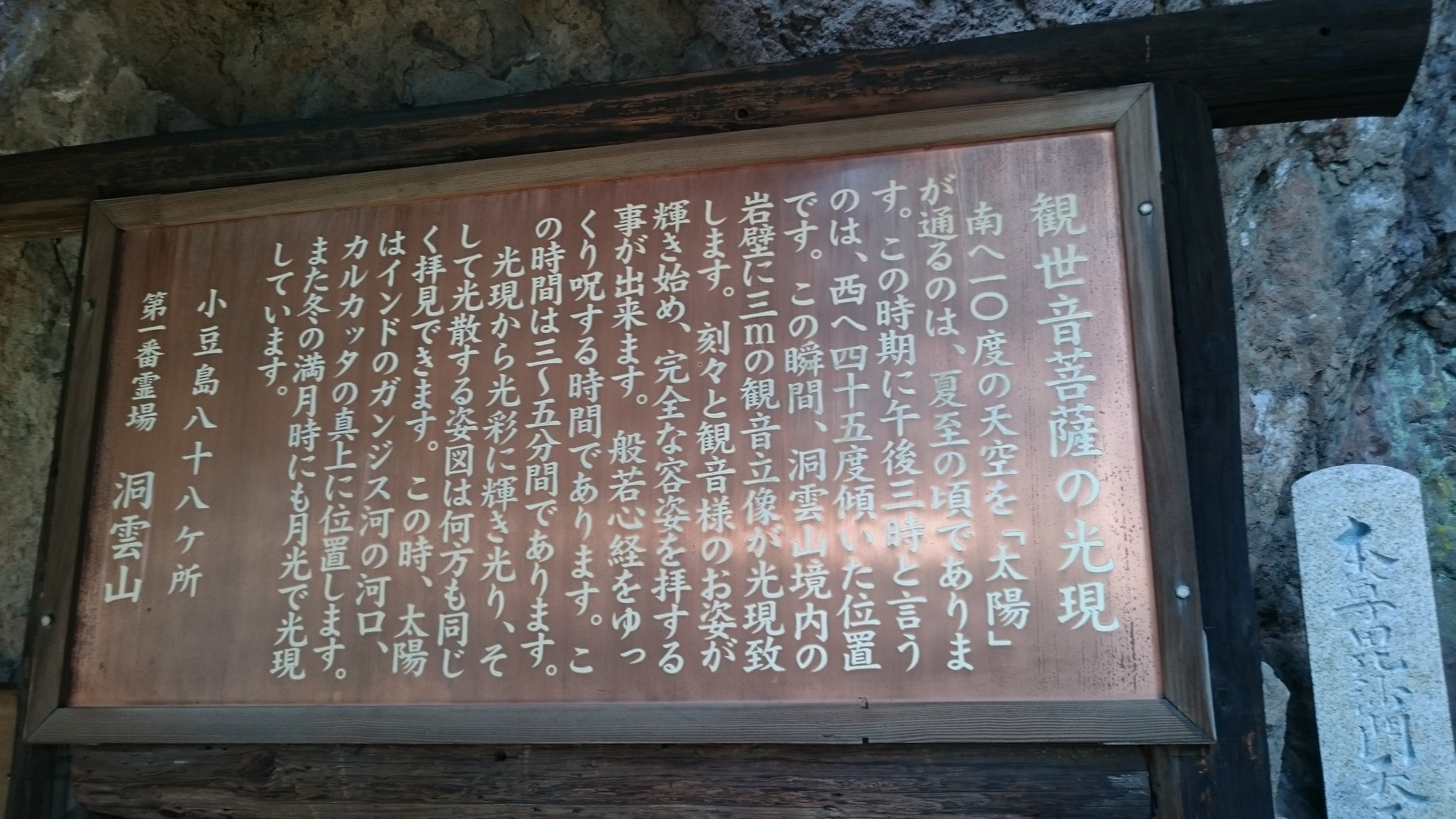The image depicts an antique-looking sign with a dark brown wooden frame encasing a copper-colored board. The board, aligned vertically, features 21 columns of Japanese text written in white characters. The first two columns on the left are somewhat spaced apart from the rest and from each other, while the last two columns on the right are larger, with a small gap between the rightmost column and the one next to it. The background behind the sign includes a variety of dark-colored stones, evoking the appearance of a cave entrance. To the right of the sign stands a stone pillar with more Japanese characters engraved in it. The sign's metallic surface is slightly shiny, with some black spots scattered across it.